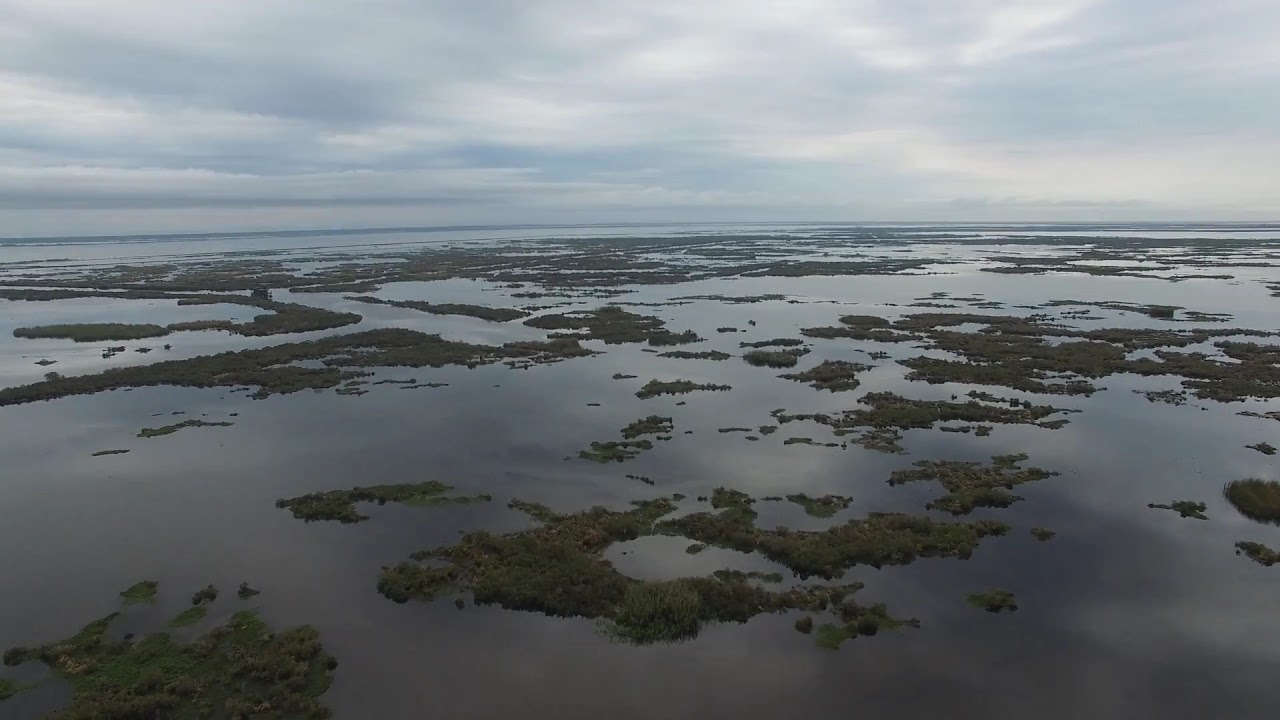The image is a panoramic, top-down photograph, likely taken from a drone or helicopter, showcasing an expansive estuary characterized by marshland. The foreground features a vast body of water that extends up to the bottom two-thirds of the photo, interspersed with patches of land and greenery that resemble small, deserted islands. This marshland is dotted with plant growth, and the dark green patches may include moss or low vegetation. The scene is set under a predominantly cloudy and overcast sky, with shades of gray and dark blue dominating the horizon. Though the distance fades into a grayish-blue expanse, possibly indicating the presence of an ocean or larger bodies of land, the overall atmosphere is one of desolation and tranquility, devoid of any human structures.